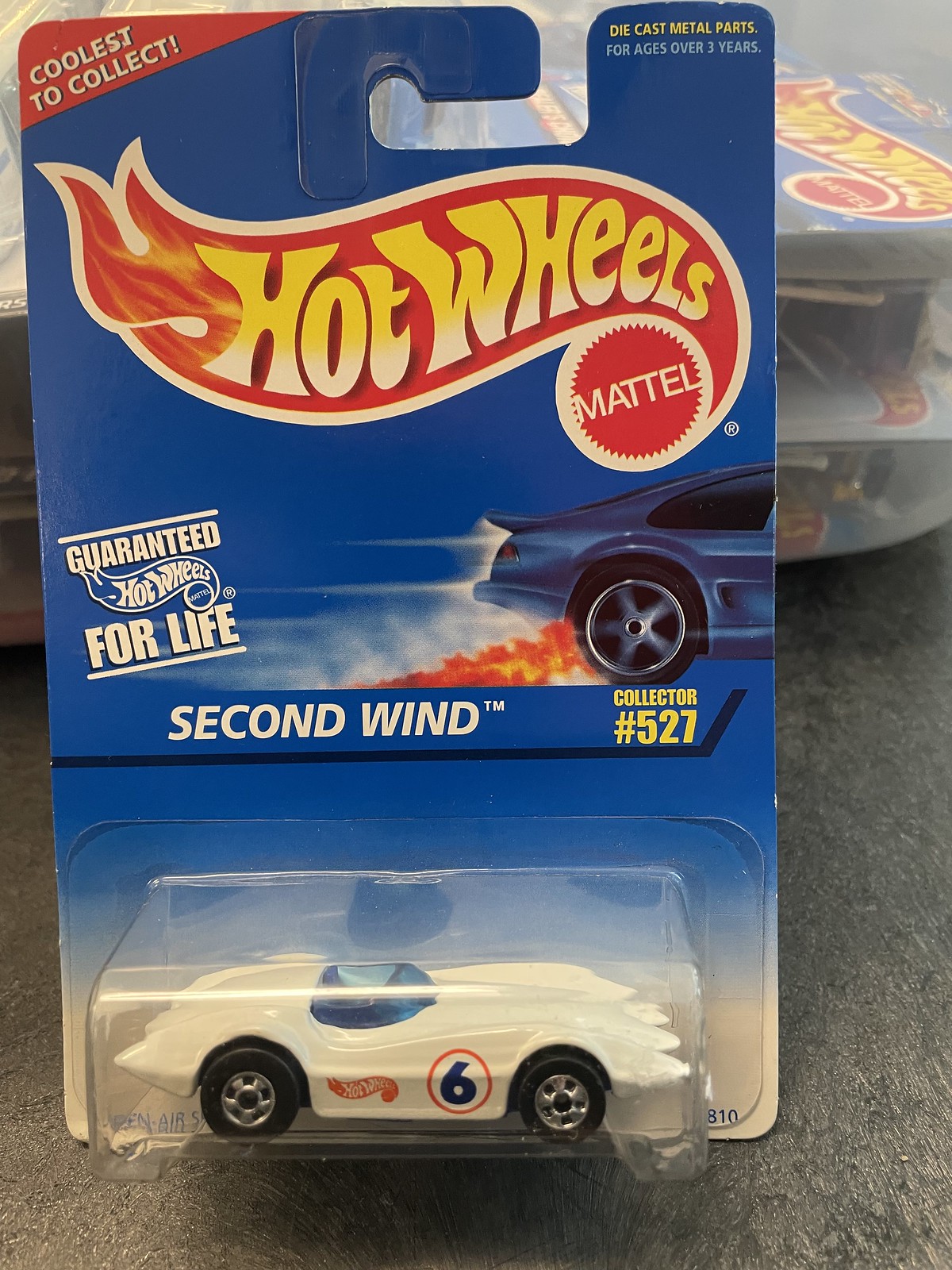The photograph captures an unopened Hot Wheels car by Mattel, propped up against a clear container of other Hot Wheels cars on a black tabletop. The car, named "Second Wind" with collector number 527, showcases a sleek white body resembling a Corvette, featuring blue-tinted windows and designed as a single-seater sports vehicle. It sports the number 6 in blue within an orange circle on its side, along with the iconic Hot Wheels logo in yellow fading to white with a red background. This older collectible is encased in a signature blue and clear plastic packaging that is glued to the cardboard backing. The packaging displays various distinctive labels: "Guaranteed for Life" on the left side, "Coolest to Collect" in the top left corner, and "Die Cast Metal Parts for Ages over 3 Years" in the top right corner. The Hot Wheels branding is prominently displayed with the classic flame-like design, using red, yellow, and white colors against the blue backdrop.